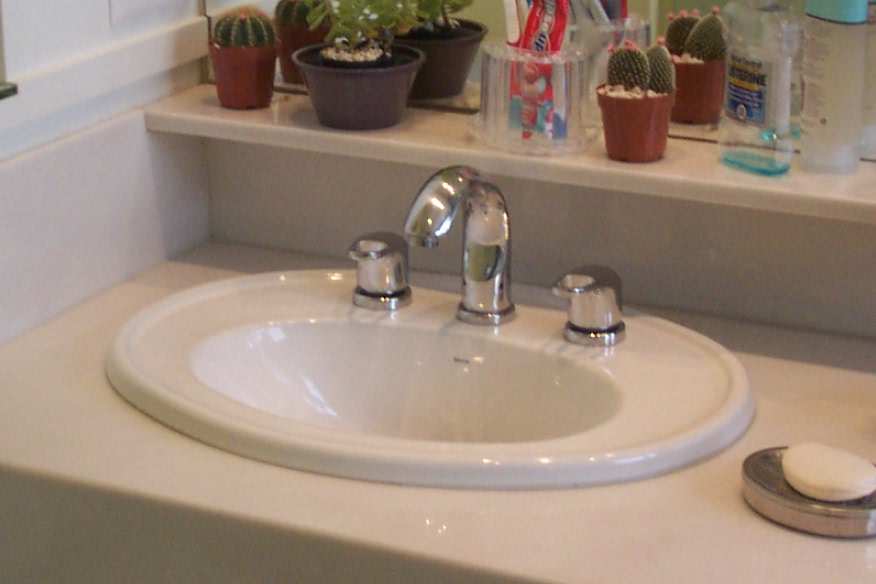This photograph captures a well-organized bathroom sink unit, featuring a small, built-in basin in a light pink cream color. The sink, embedded within a spacious countertop, is equipped with a central mixer tap having separate controls for hot and cold water. Atop the counter lies a soap dish containing a bar of white soap, the only item placed at the same level as the sink.

Above the sink is a shelf, seamlessly integrated into the unit, which is adorned with various items. On the left, a small cactus in a brown plastic pot adds a touch of greenery, accompanied by another succulent plant. Centrally, a transparent container holds toothbrushes and toothpaste, ensuring easy access. To the right, another cactus stands beside an almost empty bottle of mouthwash, possibly Listerine, hinting at an imminent need for replenishment.

The clean and minimalist design of the bathroom is accentuated by the reflection of the shelf in the mirror behind, completing the serene and orderly appearance of this space.